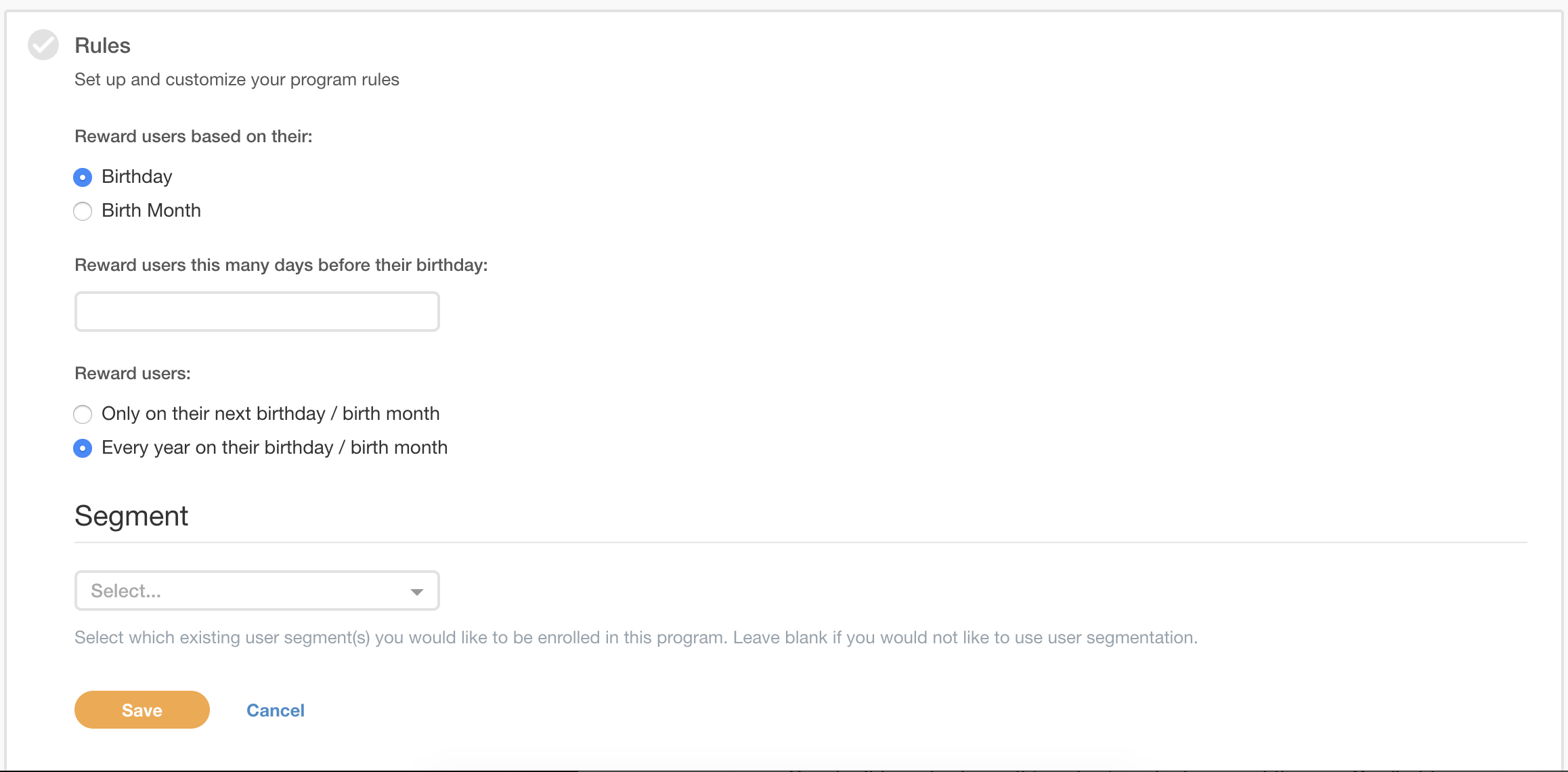The image displays a webpage dedicated to setting up and customizing program rules. At the top, in bold text, it reads "Rules" with a grey checkbox next to it, followed by a prompt to "set up and customize your program rules." Below this, there is a section titled "Reward users based on their" with two radio button options: "Birthday" and "Birth Month." The "Birthday" option is selected, indicated by a blue circle.

Following this, there is an instruction that says, "Reward users this many days before their birthday," next to an empty input box where the number of days can be specified. Underneath, another option reads, "Reward users," accompanied by two choices: "Only on their next birthday/birth month" and "Every year on their birthday/birth month." The "Every year" option is selected, also marked with a blue circle.

Further down, there is a segment section labeled, "Select which existing user segment you would like to be enrolled in this program. Leave blank if you would not like to use user segmentation." This is accompanied by a blank dropdown box for selecting user segments.

At the bottom of the page, there are two prominent buttons: an orange "Save" button and a blue "Cancel" button. The entire page layout is set against a white background with black text, featuring various interactive elements such as radio buttons and blank input fields to enable the customization of user experience.